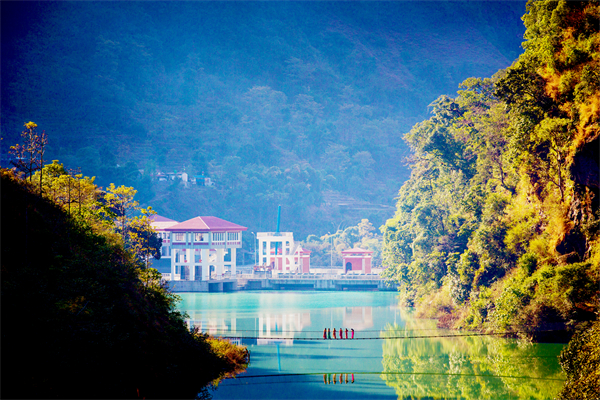The photograph captures a scenic landscape featuring a rope bridge suspended over a blue lake, connecting two landmasses densely populated with green trees. On the right side of the image, the terrain is lush with dense foliage, while the left side is dominated by a rocky hill covered with bushes. At the center of the bridge, six people are visible, casting reflections in the water below. The background reveals a charming settlement with white and red-roofed buildings near the lake's edge, extending into a bay with docks. Beyond this settlement, a massive mountain covered in dense green trees rises, providing a majestic backdrop to the entire scene. The photo is taken from a distance, giving a comprehensive view of the picturesque setting.